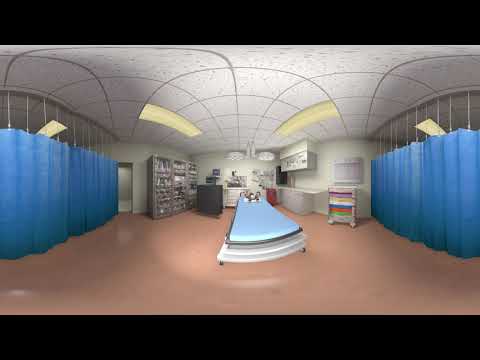The image is an interior shot of what appears to be an infirmary room, possibly within a hospital or doctor's office. At its center, an elevated medical bed stands out, featuring a white base on black wheels and a light blue mattress with a rectangular white pillow. The floor has a shiny, peachy brown, or tannish pink finish.

Blue curtains hang from white strings on both sides of the room, attached to rails mounted on the ceiling. The ceiling itself is composed of large, rectangular white panels segmented by grey lines, featuring several rectangular fluorescent lighting fixtures that illuminate the room. 

On the right side of the image, there’s a small cabinet with multiple drawers in various colors—purple, yellow, white, blue, red, and green. Above the drawers, another small cabinet is mounted on the wall. Below this arrangement, a countertop extends with additional cabinets hanging on the wall above it. A black cabinet is also visible against the wall, along with several shelves that have a glass barrier, filled with unspecified items.

On the left side, another black cabinet and a large shelving unit can be seen, though the contents are not clearly discernible. A door is open near this area. From the ceiling, designer lights dangle, and behind the treatment bed, there are additional cabinets, including a red box attached to the wall. The overall setting suggests a functional, well-equipped medical space centered around patient care.